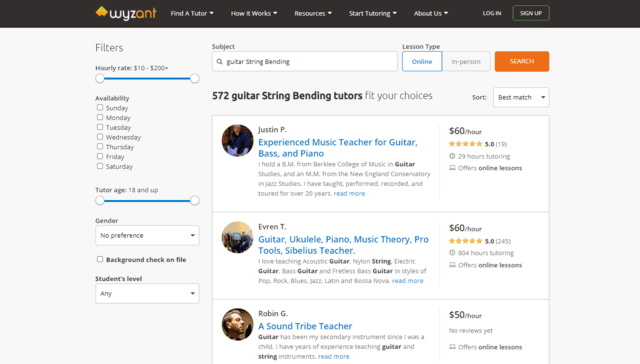This image is a screenshot from the tutoring website Wyzant, identifiable by its distinctive logo on the left, which features a diamond shape in orange and yellow hues. The logo displays "Wyz" in white letters and "ant" in gray. To the right of the logo, there is a navigation menu with options labeled "Find a Tutor," "How It Works," "Resources," "Start Tutoring," and "About Us." Additionally, there are buttons for "Log In" and "Sign Up."

On the left side of the image, there is a detailed filter panel to customize search criteria for tutors. The filters include adjustable hourly rates ranging from $10 to over $200 per hour. Availability options allow users to select specific days of the week—Sunday through Saturday—each accompanied by a checkable box.

Further customization options include the tutor's age, with available choices starting from 18 and above, and the ability to specify preferences for the tutor's gender, the presumption being the default is set to no preference. The panel also has an option to filter tutors based on whether they have a background check on file. Finally, users can select the student's level, with a default setting of "Any," which can be adjusted as needed.

Overall, the screenshot illustrates Wyzant’s user-friendly interface designed to help customers find the best matching tutor according to their specific requirements.